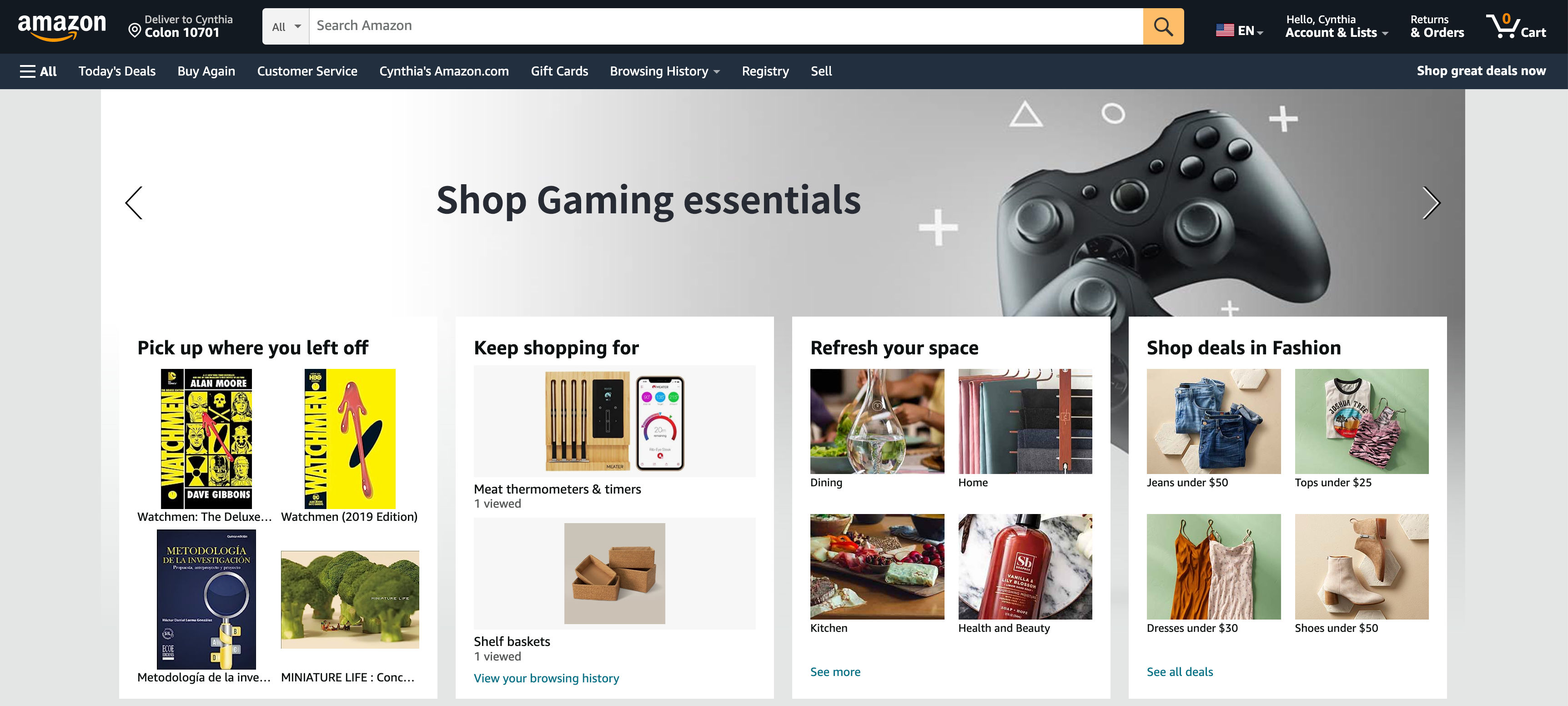In this detailed image from the popular retail site Amazon, the top left corner features the iconic Amazon logo on a sleek black header. Adjacent to the logo, customer information is displayed, reading "Delivered to Cynthia: 10701." Moving to the right, the prominent Amazon search bar is placed for easy navigation. Further to the right, the header includes personalized options: "Hello, Cynthia," "Accounts and Lists," "Returns and Orders," and a Cart button.

Below the header, a navigation bar offers quick access to various sections: "Today's Deal," "Buy Again," "Customer Service," "Cynthia's Amazon.com," "Gift Cards," "Browsing History," "Registry," and "Sell." The central portion of the page showcases a large, visually striking advertisement featuring a game controller with the text "Shop Gaming Essentials."

Beneath this ad, the content is divided into several sections. Starting on the left, a segment titled "Pick Up Where You Left Off" displays Cynthia's recently viewed items, which include an assortment of graphic novels, books, and miniatures. The middle section highlights "Keep Shopping For," showcasing items such as thermometers and baskets. On the right, the "Refresh Your Space" section advertises home goods, followed by another section promoting "Shop Deals and Fashions," featuring various clothing items.